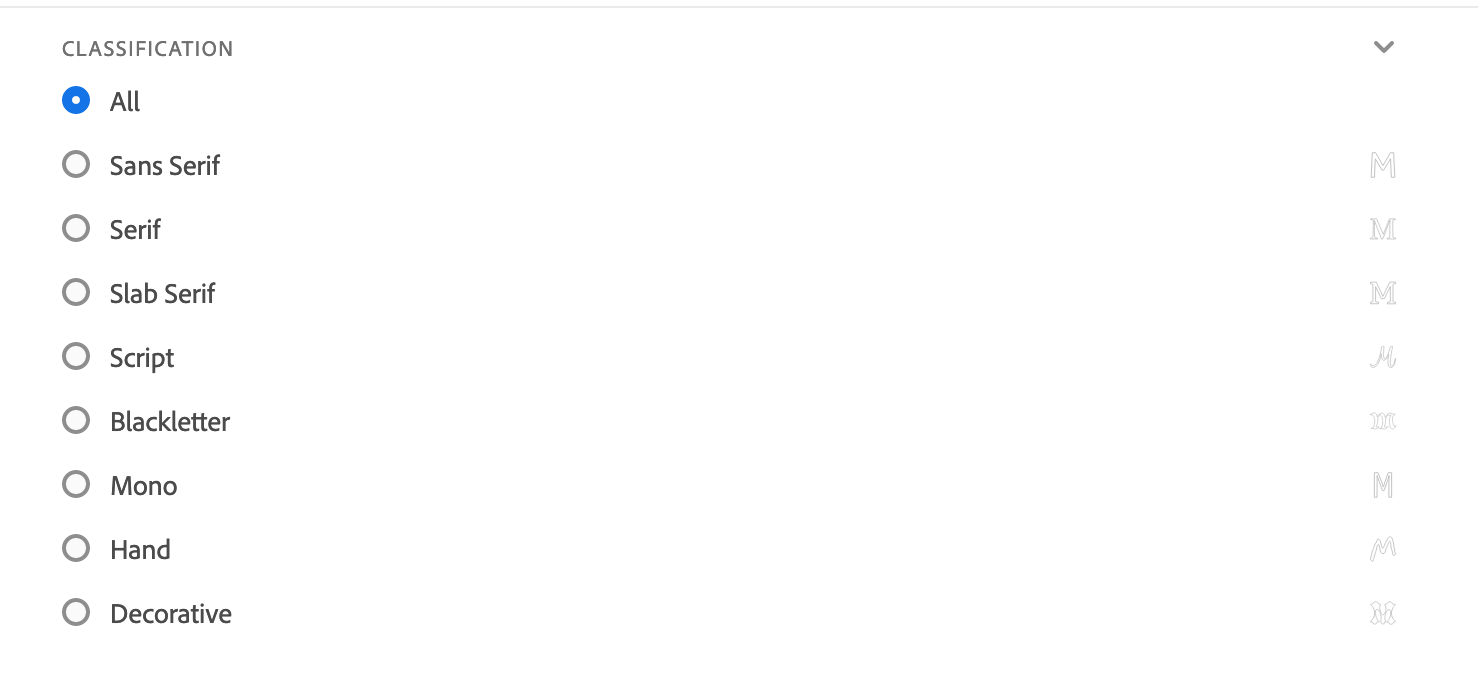The image depicts a classification screen with a white background. On the left side, there is a vertical column listing nine different font categories, each accompanied by an unchecked blue circle. The categories are: All, Sans Serif, Serif, Script, Black Letter, Monospaced, Handwritten, and Decorative.

Adjacent to each category, the letter "M" is displayed in various fonts corresponding to the category. For instance, "M" is shown in a Sans Serif font under the Sans Serif category, in a Script font under the Script category, and so forth, including Black Letter, Monospaced, Handwritten, and Decorative fonts. The Decorative font appears to be particularly creative and elaborate.

The screen appears to focus solely on font classification, presenting an orderly array of font styles for comparison. The interface is minimalist, containing few other elements besides the font categories and their respective examples. The purpose of the classification remains unclear, but the overall layout is straightforward, with no additional activities or interactive elements present on the screen.